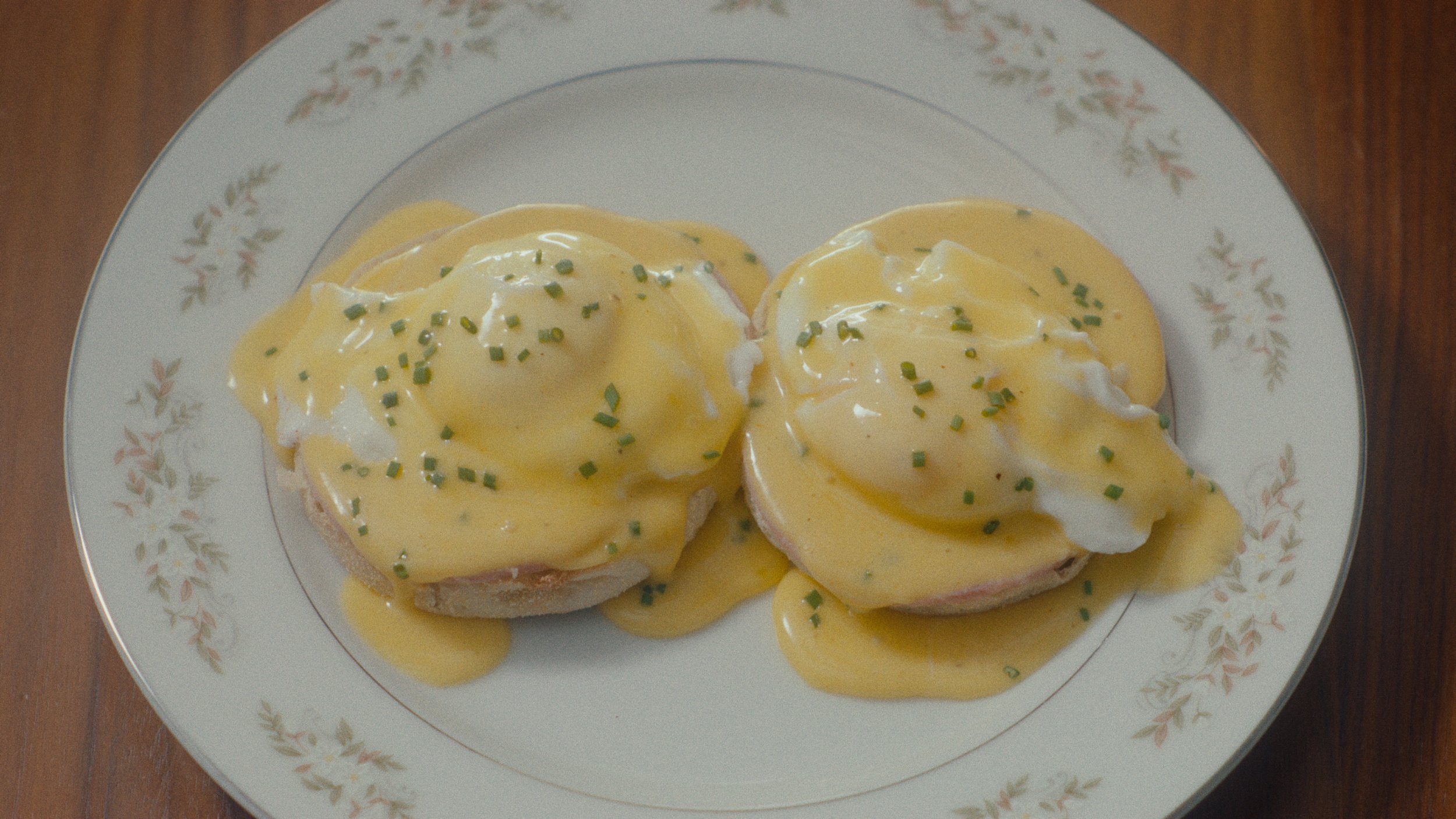The image captures a detailed view of a food dish, likely Eggs Benedict, beautifully plated on a white, circular plate adorned with faint floral designs and a thin gray border around the edge. The plate rests on a stained wooden table, hinting at a homely or rustic indoor setting, likely illuminated by artificial light, which gives the photograph a muted, understated tone. The dish consists of two servings of Eggs Benedict, each featuring an English muffin base and a poached egg, generously draped in rich hollandaise sauce. The sauce is speckled with finely chopped green onions or similar green seasoning, adding a delicate touch of color to the golden-yellow sauce. Though the ingredients and effort behind the preparation are evident, the overall presentation is sophisticated and meticulously arranged.